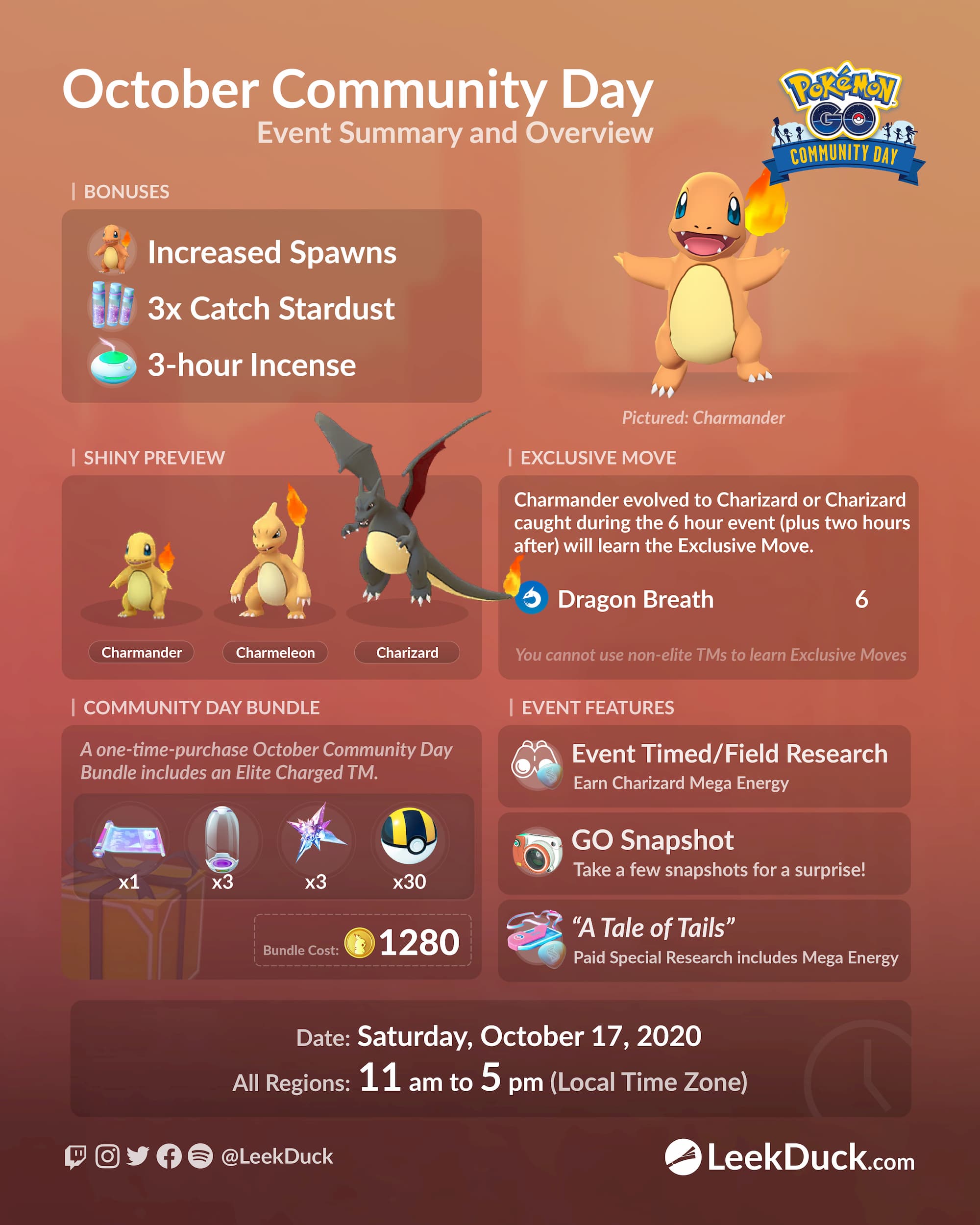This digital image features a vibrant background that transitions from a light orange at the top to a dark red at the bottom. In the top left corner, large white text reads "October Community Day," with a smaller subtitle below stating "Event Summary and Overview" in white. The top right corner displays the "Pokemon" logo in cartoon-style yellow lettering with a blue outline, accompanied by blocky blue text "GO" beneath it. Below this, a blue banner with yellow all-caps text announces "Community Day."

On the left side of the image, an orange, cartoonish, dragon-like creature known as Charmander is depicted. Charmander is holding a flame in its left hand and has an eggshell-white belly. Below Charmander, italicized white text reads "Pictured: Charmander."

Adjacent to Charmander, a translucent black rectangle with rounded corners contains event information. Above this rectangle, a white separator bar introduces the word "Bonuses" in white. The rectangle itself presents various icons and text detailing specific event bonuses: 
- A light gray circle featuring Charmander with the text "Increased Spawns" to its right.
- Three blue and purple pillars icon with the text "3× Catch Stardust" beside it.
- A white and green rounded object emitting smoke, with "3 Hour Incense" written next to it.

Additional tiles with similar icons and white text provide further event bonuses throughout the rest of the image. In the bottom right corner, white text credits the source as "LeekDuck.com" with "L E E K D U C" spelled out beneath it.